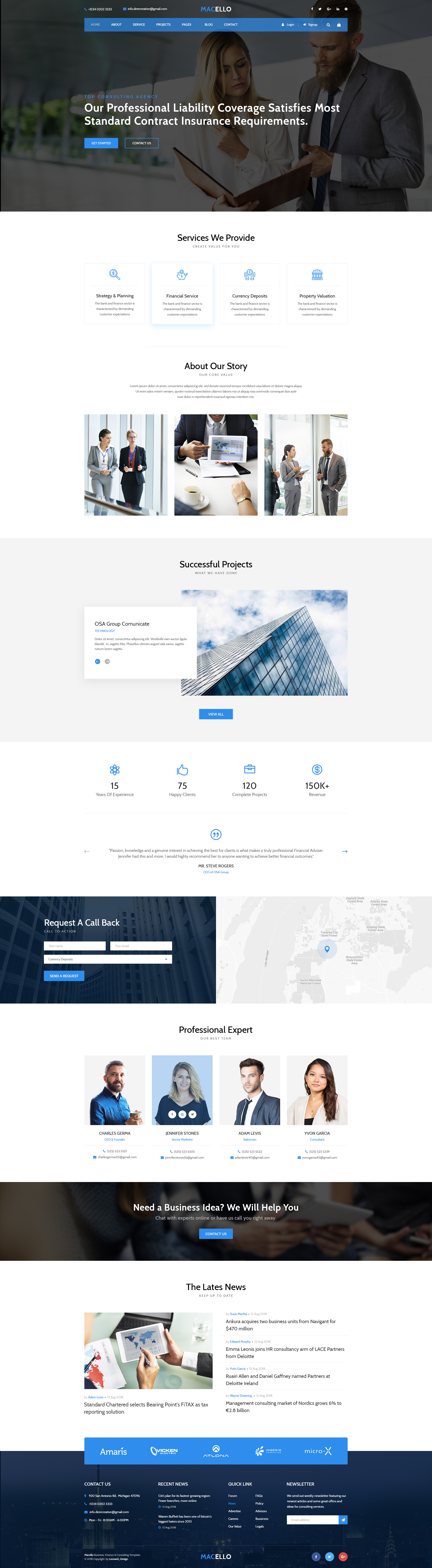**Detailed Caption:**

The screenshot appears to be from the website of a consulting agency named Macello. At the top of the page, against a blue banner, the company's name "Macello" is prominently displayed, accompanied by a phone number and an email address for contact. Links to their various social media profiles are also present.

The primary navigation menu includes options for Home, About, Services, Products, Pages, Blog, and Contact. There are also buttons for users to Log In or Sign Up.

In bold text, the site proclaims itself as a "Top Consulting Agency" and assures that their professional liability coverage meets most standard contract insurance requirements. Below this, there are call-to-action buttons labeled "Get Started" and "Contact Us."

A section titled "Services We Provide" emphasizes creating value for clients through offerings such as Strategy and Planning, Financial Services, Currency Deposits, and Property Valuation.

The "Our Story" section features imagery to enhance the narrative, starting with a photograph of two women walking together, followed by an image of someone pointing at something, likely demonstrating an explanation, and concluding with a snapshot of three people—two men and one woman—engaged in discussion.

Under the "Successful Projects" segment, projects completed by Macello are highlighted. The first project mentioned is the "OSA Group Communicate," accompanied by an upward-looking photo of a building. A clickable link titled "View Them All" invites users to explore more.

Statistics displayed on the site boast 15 years of experience, 75 happy clients, 120 complete projects, and a revenue of over 150K.

The website also includes a "Request a Callback" call-to-action form where users can input their name and other relevant information before submitting a request.

At the bottom of the page, the "Professional Experts" section introduces team members Charles, Jennifer, Adam, and Yvonne. A motivational statement "Need a business idea? We will help you" is prominently featured followed by the "Latest News" segment, which keeps visitors updated with recent happenings related to the company.